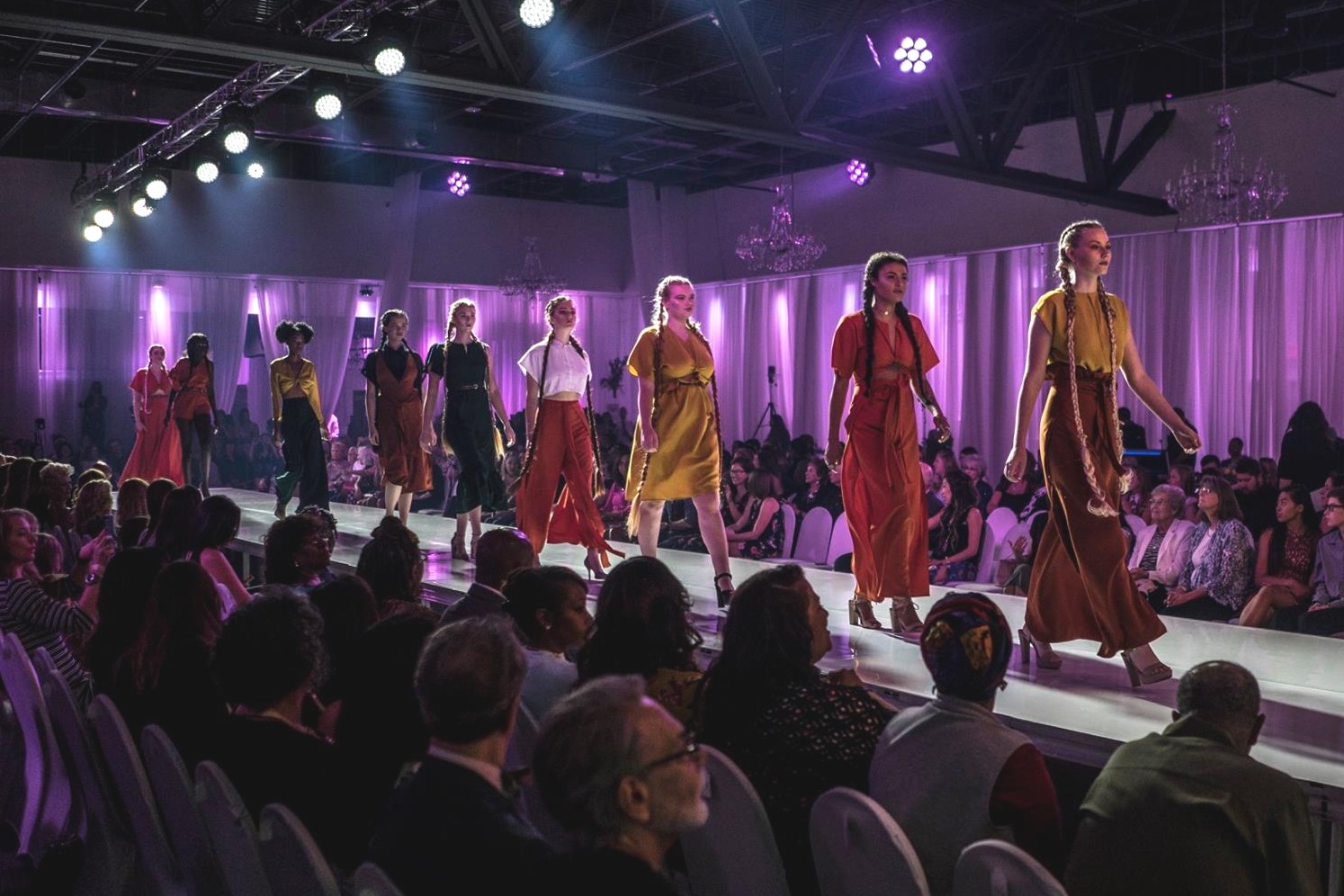This color photograph, captured in landscape orientation, showcases an interior scene of a fashion show runway, dramatically extending from the center left of the image towards the bottom right corner and widening in perspective as it approaches the foreground. Lined with viewers on both sides, the runway sits approximately 30 inches above the audience, who are intently watching the procession of models. The spotlighted stage features about nine female models adorned in various dresses, elegantly parading down the catwalk. 

At the forefront, one striking model is dressed in a captivating ensemble of a gold short-sleeve shirt paired with a long burgundy dress reaching her ankles. She boasts extraordinarily long, gold-braided pigtails extending down to her knees. Each model in the line contributes to the visual spectacle, with another notable model behind her wearing a red dress with elbow-length sleeves, and following her, another model in a gold dress stopping just above her knees. Overhead, an array of spotlights illuminates the scene, casting sharp, dramatic shadows, enhancing the representational realism style of the photograph, while purple floodlights bathe the surrounding curtains, adding to the glamorous ambiance of the event.